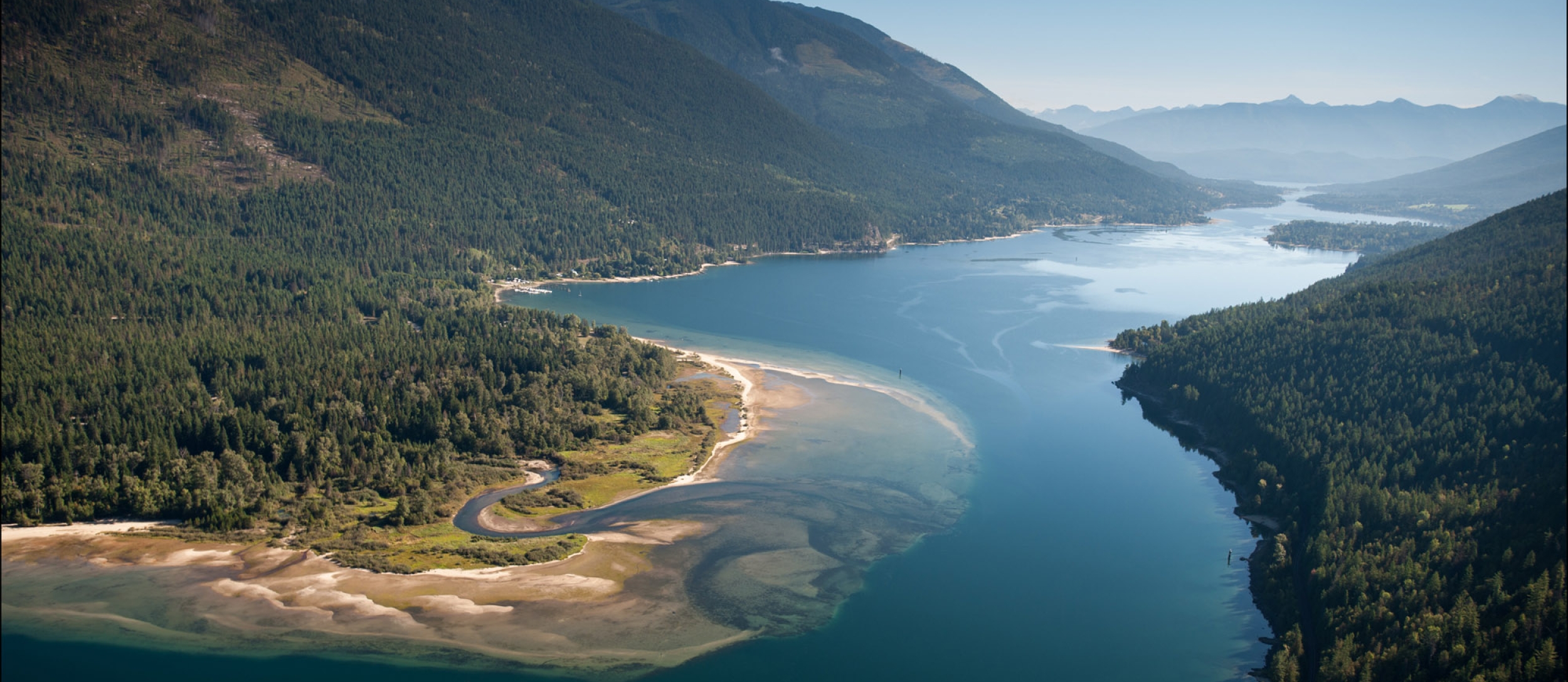This aerial photograph captures a stunning scenic landscape showcasing a meandering river that winds through a lush, forested valley. The river, a deep and reflective dark blue, stretches from the expansive foreground, narrowing into the distance where it meets a backdrop of towering, clear blue mountain ranges. On the left bank, a sandbar extends halfway across the river, bifurcated by a small creek flowing into the dense forest. This sandbar is part of a peninsula that juts into the river, adding a dynamic, natural formation to the scene. The surrounding mountainsides are blanketed in dense, vibrant green trees, lending a sense of tranquility and peace to the image. The waterway shows variations in color, potentially suggesting foam or differing water depths, adding richness to its appearance. Further back, the river curves and flexes, disappearing into the horizon where it merges with a distant, majestic mountain range under a clear blue sky. This beautifully detailed and photorealistic image exudes natural serenity and picturesque beauty.